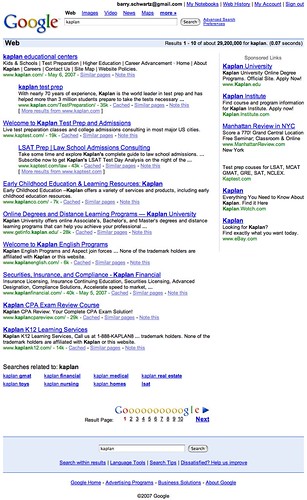A Google search results page is displayed where the user has typed "Kaplan" into the search bar. The iconic Google logo appears prominently at the top, showcasing its multicolored letters: a blue capital "G," a red lowercase "o," a yellow lowercase "o," a blue lowercase "g," a green lowercase "l," and a red lowercase "e." Below the search bar, the top search result is for "Kaplan Educational Centers." This entry is followed by a link to "Kaplan Test Prep and Admissions," offering services like LSAT Prep and Law School Admissions Consulting. Another link presents resources related to Early Childhood Education and Learning, labeled simply as "Kaplan." Each of these results is accompanied by a clickable green URL link. On the right-hand side of the results page, there are suggested sponsored links for "Kaplan University," "Kaplan Institute," "Manhattan Review," and "New York City," further extending the range of Kaplan-related search outcomes. The search results continue down the page with various entries related to the Kaplan brand and its educational services.